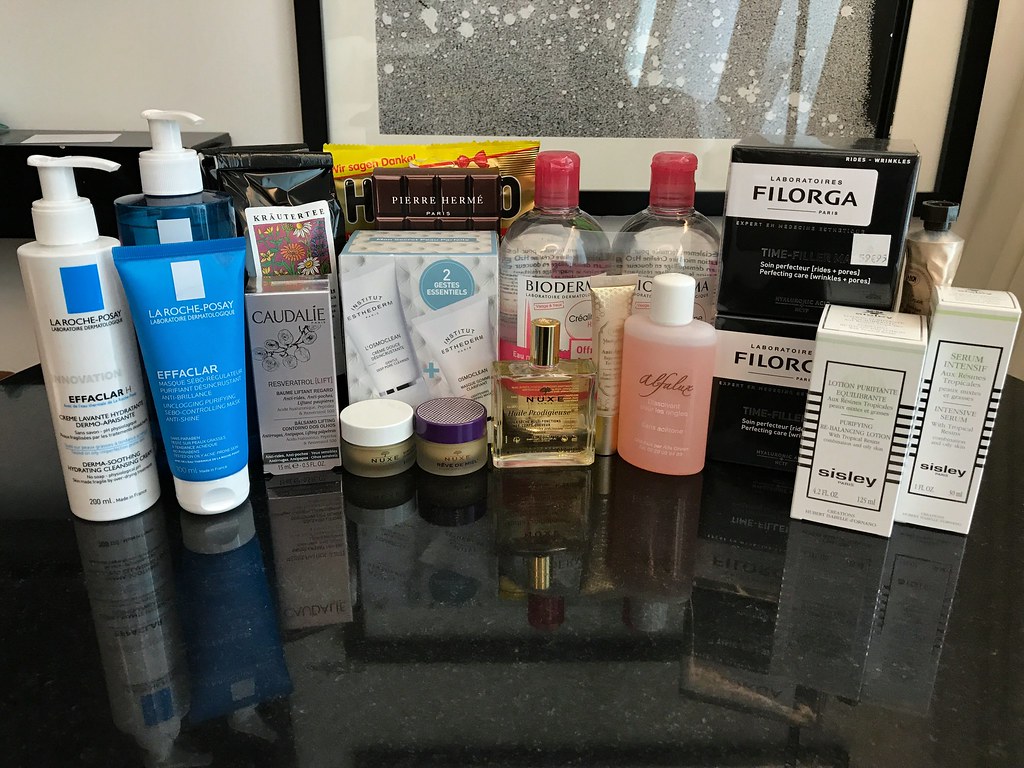A visually appealing arrangement of luxury skincare products is meticulously displayed on a wall shelf. To the left, two La Roche-Posay bottles dominate the scene, one in white and the other in blue, each equipped with a convenient white pump. Adjacent to them sits a blue squeeze tube from the same brand, suggesting a cohesive collection. Next in line is a sophisticated silver box from Caudalie, featuring the Resveratrol-Lift range, although further details remain indistinct.

Continuing the sequence, a prominently displayed box showcases two white tubes, hinting at additional skincare essentials. In the foreground, two charming, frosted glass tubs of Nuxe lip balm attract attention with their pastel lids—one white and one purple—revealing the yellow balm inside. Moving right, a sleek rectangular glass bottle of oil, also from Nuxe, adds a touch of elegance to the display. Behind it, two plastic bottles of Bioderma are filled with clear liquid and capped with white tops, their labels gleaming with brand recognition.

The arrangement proceeds to feature two black boxes stacked atop one another, bearing the inscription "Laboratoires De Lorgia" in minimalist white font. Completing the curation, two white boxes with contrasting black lettering signify products from Sisley: a Purifying Rebalancing Lotion and an Intensive Serum.

Above this luxurious assortment hangs a sophisticated black-and-white framed photograph or artwork, encased in a simple yet elegant black frame, adding a touch of artistry to the meticulously curated space. This lineup of beauty products suggests a recent haul, reflecting a sophisticated and discerning skincare enthusiast's taste.